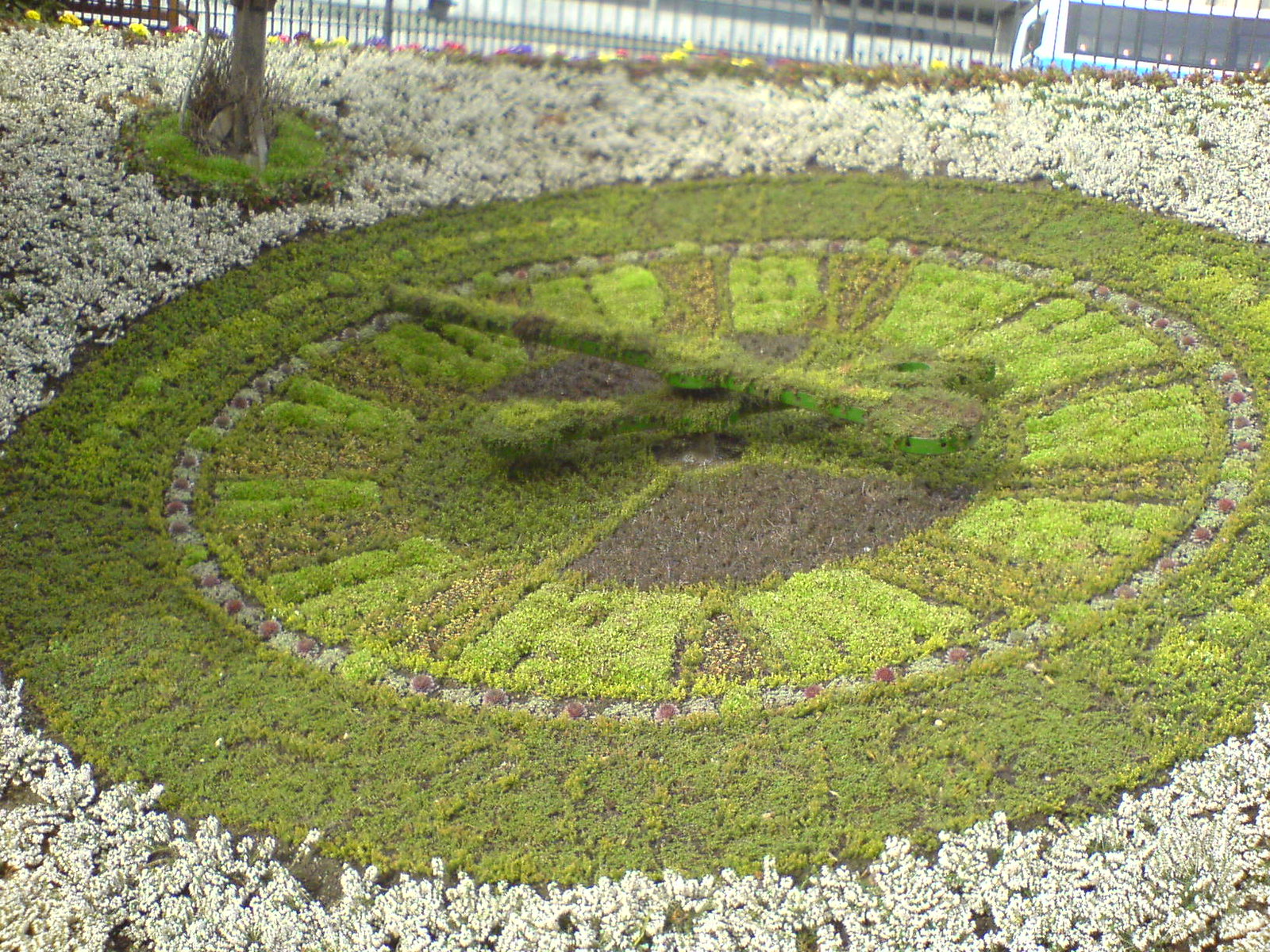This is an aerial-view color photograph of an intricately designed garden clock. The clock face, composed of meticulously arranged greenery, features Roman numerals formed by pruned plants. The clock hands are large, green frames covered with moss or grasses. Surrounding the clock face is a circular ring of white and lavender flowers, interspersed with purple orbs. This ring is bordered by a well-kept, vibrant grass circle. Beyond this, another ring of white flowers, possibly alyssum, encircles the garden, and in the distance, a wrought iron fence delineates the property. In the upper left corner, the shadow of a nearby tree provides contrast to the verdant scene. This beautiful display is likely part of a park or botanical garden, highlighting the union of horticulture and artistry.